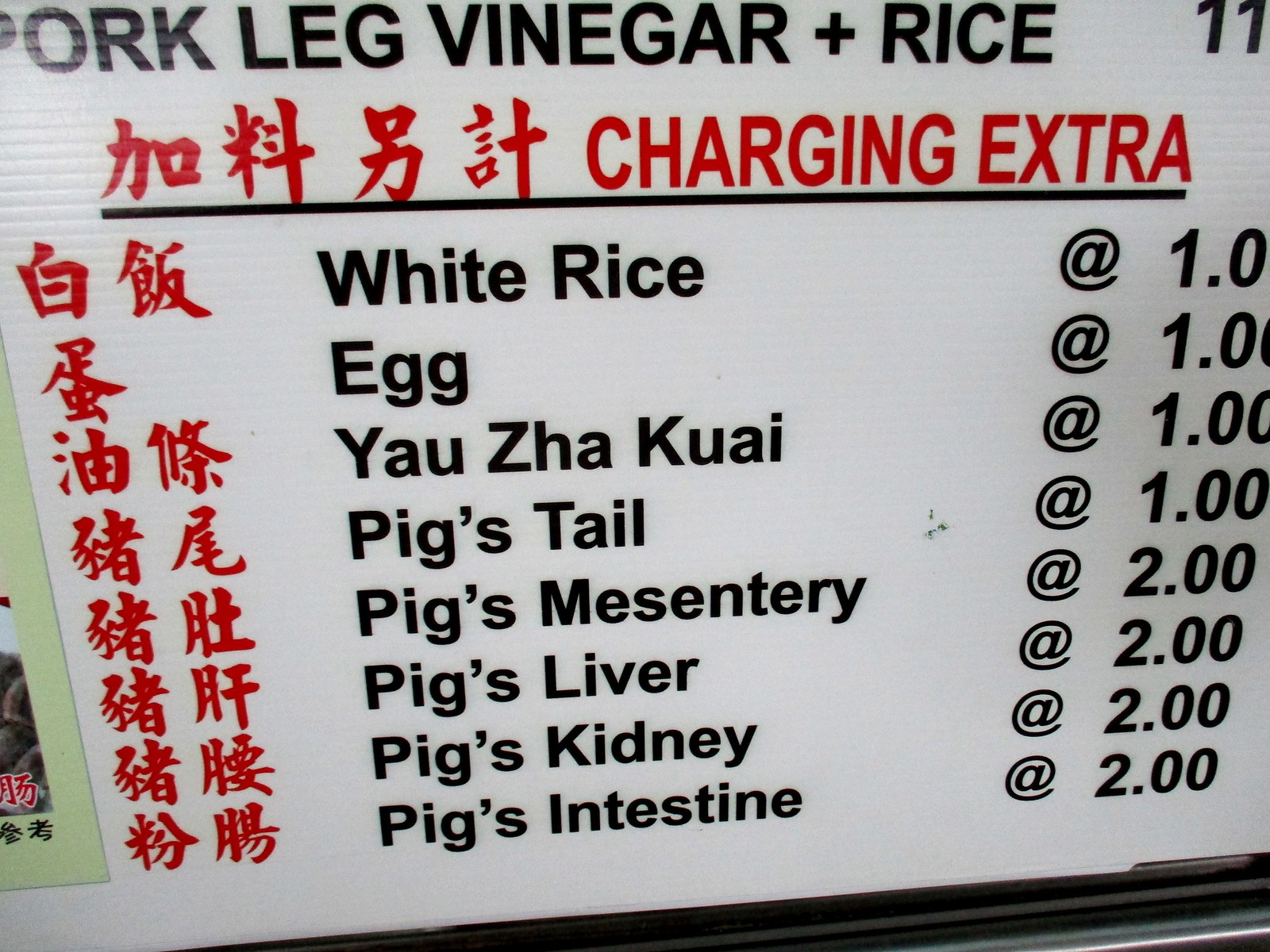This photograph depicts a white menu from a Chinese restaurant. At the top left corner, the main dish listed is "Pork Leg Vinegar plus Rice," priced at $11. Below, the menu specifies in red Chinese characters that certain add-ons come at an extra charge. The add-ons include white rice for $1, an egg for $1, yaosa (likely a transliteration for another food item) for $1, and various pig parts: pig's tail for $1, pig's mesentery for $2, pig's liver for $2, pig's kidney for $2, and pig's intestine for $2. Each item on the list is flanked by red Chinese writing, providing an authentic feel to the menu and indicating the additional costs for these extra items that can be added to the main meal or possibly other dishes.